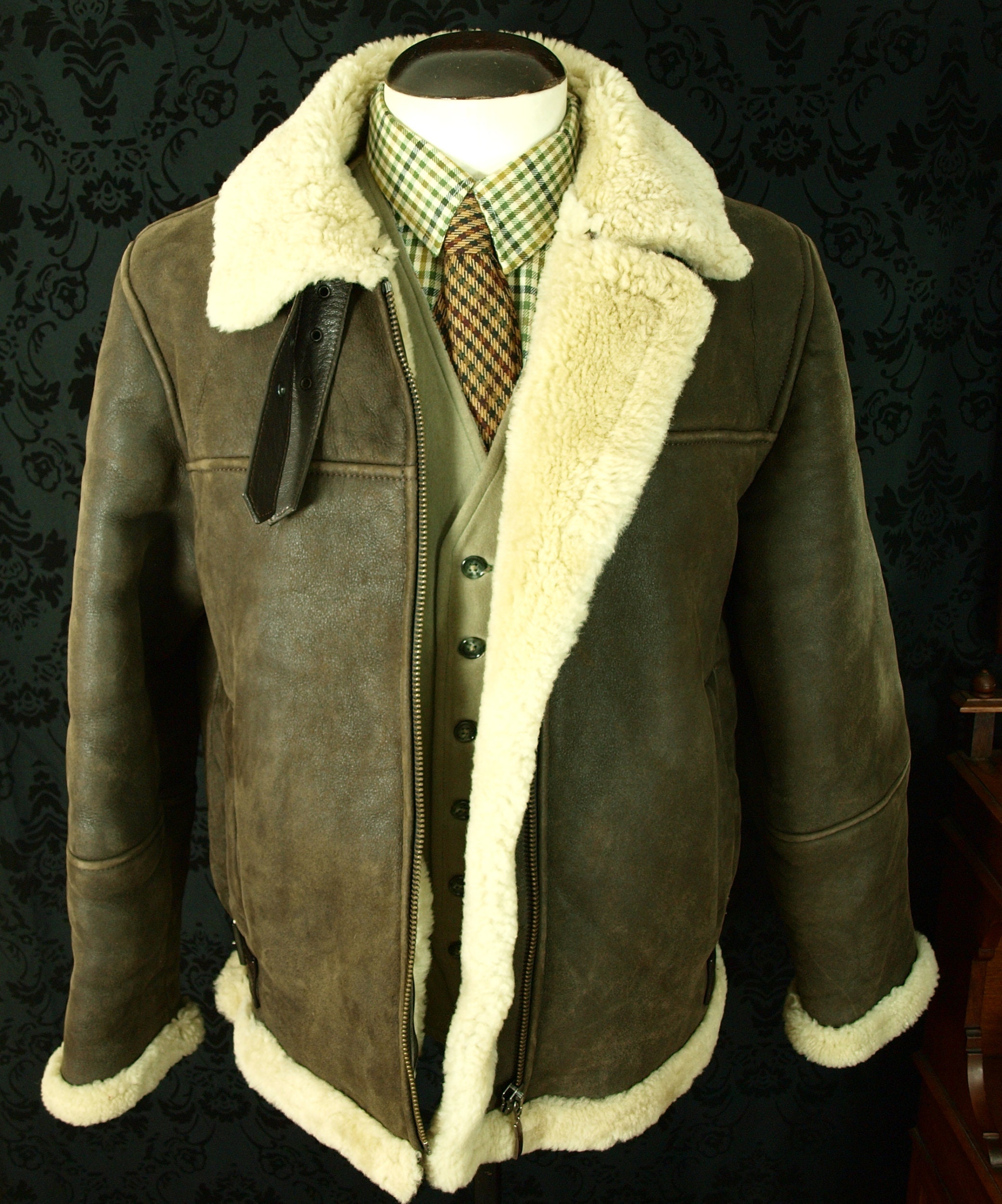The image shows a headless mannequin set against a black background adorned with an old-style floral pattern in black. The mannequin is dressed in a highly detailed, layered outfit. The innermost layer is a checkered shirt in hues of dark blue, yellowish tan, and green, paired with a matching checkered tie featuring maroon, dark blue, and green on a khaki background. Over this, the mannequin wears a fully buttoned tan vest. Completing the ensemble is a dark brown, World War II-era bomber jacket. This leather jacket is lined with plush sheepskin, visible at the wide collar, lapel, waistband, and the cuffs of the sleeves. The jacket includes pockets on either side, each equipped with zippers. The intricate textures and colors of the outfit stand out vividly against the ornate, floral-patterned wallpaper, providing a stark yet complementary contrast. Next to the mannequin, the edge of a wooden piece of furniture, possibly a desk, is visible.